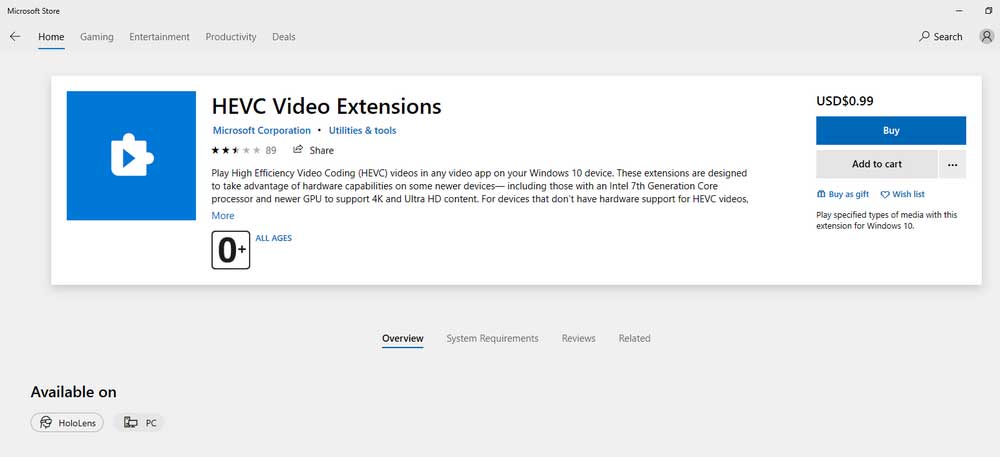The screenshot captures the window of the Microsoft Store as displayed on a desktop computer screen, with an off-white background. In the upper-left corner, the title "Microsoft Store" is prominently written in black. Below the title, a navigation menu features the following options: Home, Gaming, Entertainment, Productivity, and Deals, with the "Home" option currently selected and underlined in blue.

The main window beneath this menu is a long rectangular section with a white background. On the left side of this section, there is a blue square containing a play button icon. To the right of this icon, in black text, it reads "HEVC Video Extensions." Directly below this, in blue text, it states "Microsoft Corporation . Utilities & tools."

On the far right side of the section, the price is listed as "$0.99 USD" in black text. Below the price, a blue "Buy" button is prominently displayed, inviting users to purchase the extension.